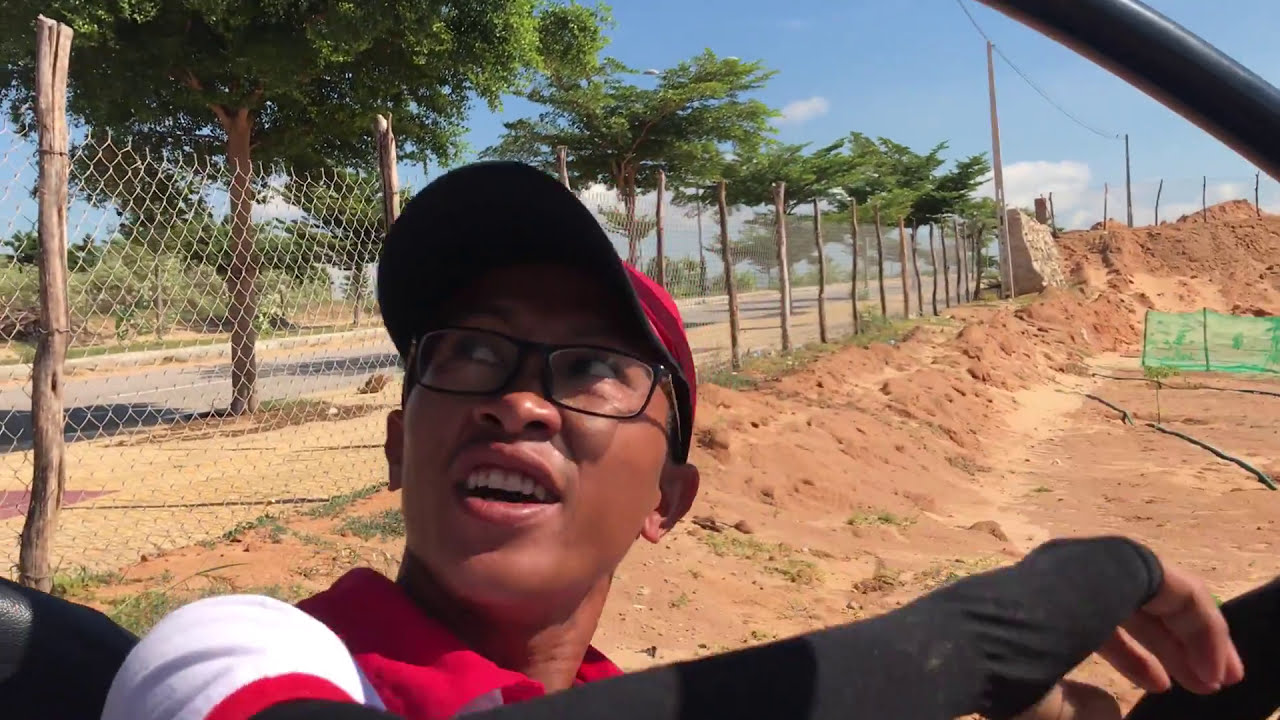In this outdoor setting, a young black man, possibly biracial, sits in a dirt area, looking up towards the upper left with an expression that suggests surprise or shock. His body is partially twisted over his right shoulder, enhancing his upward gaze. He wears a red baseball cap and black rectangular-framed glasses, accompanied by a red, black, and white collared polo shirt. His arm is positioned in front, with fingers visible as it arcs down to the right. 

The background features a sterile-looking, bare dirt terrain shaped like a bowl, surrounded by a chain link fence. Beyond the fence, there is a row of small, uniformly planted trees, approximately 20 feet in height, lining a road. Above, the sky is a clear blue with a few scattered white clouds, indicating a sunny day.